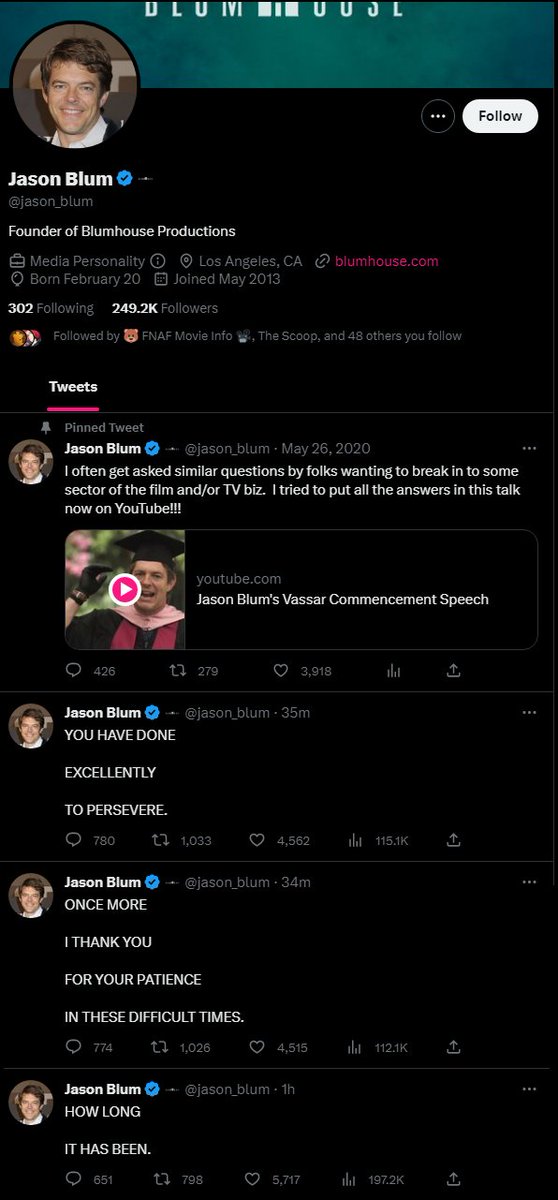The rectangular image displays a screenshot of someone’s Twitter profile, showcasing a series of their posts. The top of the image features a gradient green banner, which transitions from a lighter green in the center to a darker, spotty green towards the edges. Positioned in the middle of this banner is white text that reads "Blum House." Partially obscuring the top left portion of the banner is the user's profile picture, which is circular and depicts a man dressed in a collared shirt with the top button undone, layered with a black jacket.

Below the profile picture is the user's name in white text, "Jason Blum," followed by his username in gray text, "@JasonBlum." Additionally, a description under his username indicates that he is the founder of Blumhouse Productions. Continuing under this description, there is further gray text listing his occupation as a Media Personality based in Los Angeles, CA, along with his website, “Blumhouse.com,” his birth date, “born February 20,” and the date he joined Twitter, “joined May 2013.”

The profile statistics beneath this information reveal that Jason Blum is following 302 accounts, has 249.2K followers, and is followed by "FNAF Movie Info," "The Scoop," and "48 others you follow." The section following these details displays various tweets made by Jason Blum. The top post in this section is highlighted in white text.